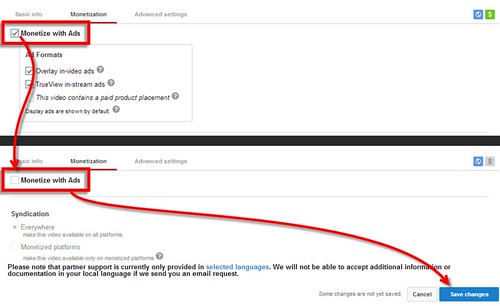### Detailed Descriptive Caption

The image shows a predominantly white screen with black text, featuring various annotations in red. It appears to be a monetization settings page on a digital platform. At the top of the screen, there is a gray, horizontal navigation bar with tabs labeled "Basic Info," "Monetization," and "Advanced Settings." The "Monetization" tab is currently selected.

A section of the screen displays two rectangular options labeled "Monetized with ads." The first option is circled in red and has a checkmark next to it, indicating it is selected. The second option is located below and also has a red rectangle around it, but it is not checked. A red arrow points downward from the first option to the second.

To the right side of the screen, another red arrow points to a blue button labeled "Save Changes" written in white font. Below the primary options, there is a section that lists various ad formats: "All ad formats," "Overlay in-video ads," "TrueView in-stream ads," and "Sponsored cards." Checkmarks indicate that "Overlay in-video ads" and "TrueView in-stream ads" are selected. Below these, there’s an option for "Video contains a paid promotion," which is not checked.

At the bottom, there appears to be a text indicating some ads' default settings, partially obscured by a horizontal black line passing through the middle of the screen. This line seems to be an annotation or divider that separates different sections of the content.

Overall, the annotations and highlighted elements suggest that this is an instructional or educational screenshot guiding users through the monetization settings of the platform.